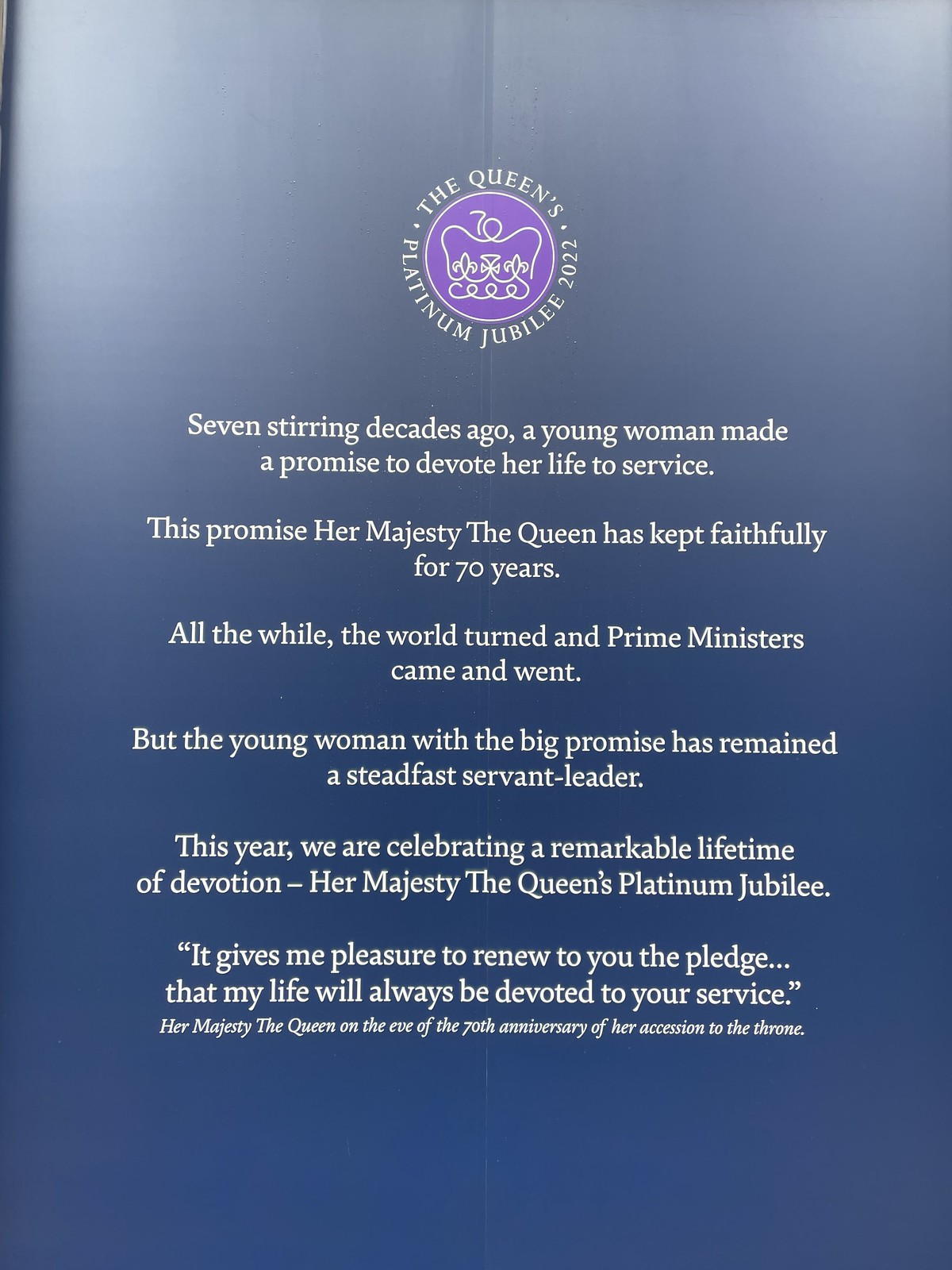This image features a scanned or digitized flyer, set against a glossy royal blue background, commemorating the Queen's Platinum Jubilee 2022. At the top of the flyer, a regal purple circle encloses an intricate white insignia, which appears to be the Queen’s crown, creatively symbolized with the numbers '7' and '0' representing her 70 years of reign. Encircling this emblem, the text reads "The Queen's Platinum Jubilee 2022". Below this, a series of poignant lines are written to honor the Queen's 70 years of unwavering service. It begins with, "Seven stirring decades ago, a young woman made a promise to devote her life to service. This promise Her Majesty the Queen has kept faithfully for 70 years. All the while, the world turned, and Prime Ministers came and went, but the young woman with the big promises remained a steadfast servant leader." The text continues, celebrating "a remarkable lifetime of devotion," and features a quote from the Queen herself on the eve of her 70th anniversary, "It gives me great pleasure to renew to you the pledge that my life will always be devoted to your service." This quote is attributed to "Her Majesty the Queen".